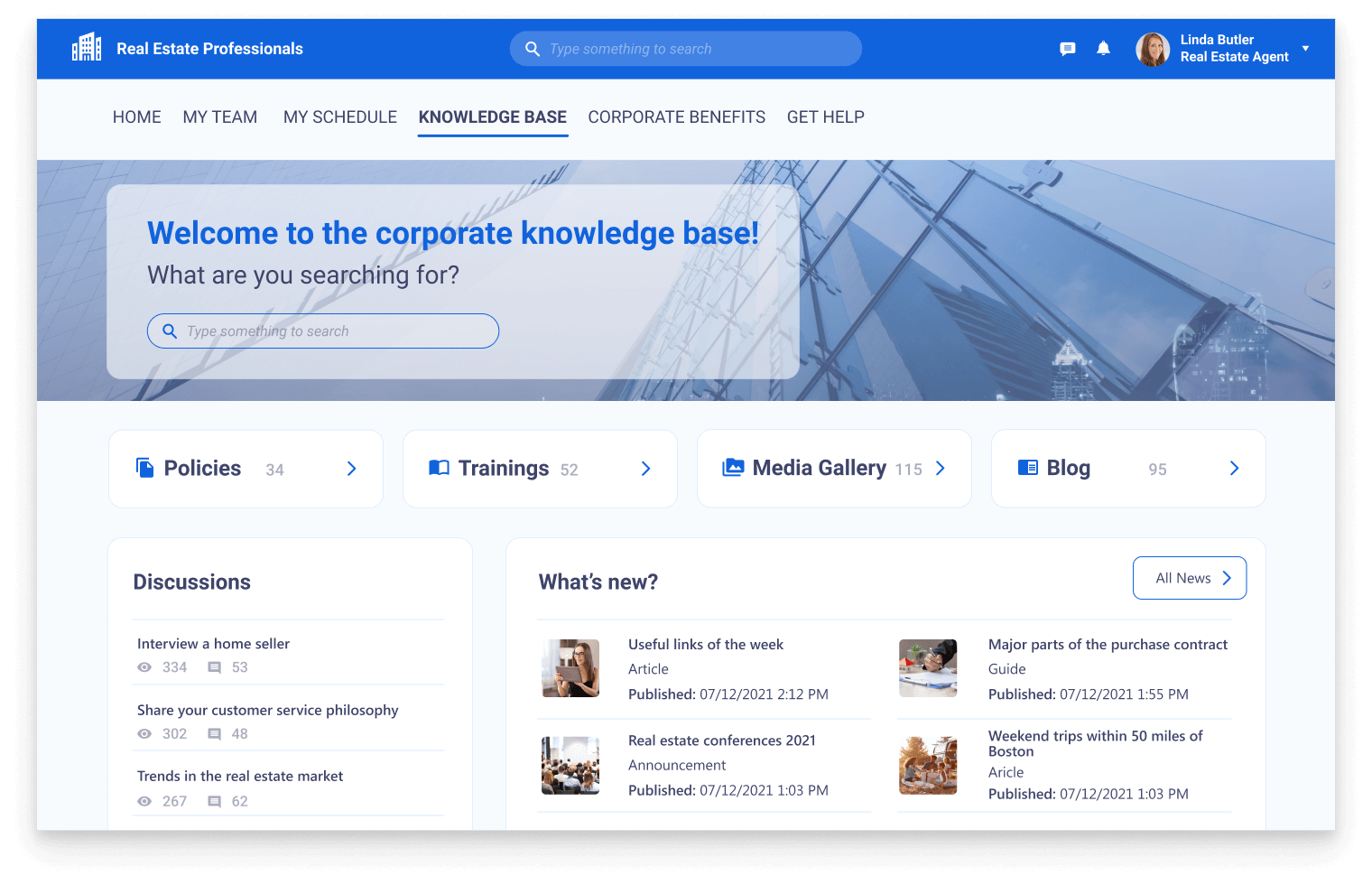The image is a screenshot of a real estate website. At the top left, a blue bar displays the text "Real Estate Professionals." In the center of this bar is a search bar, while the right side features several icons: a chat icon, a bell notification symbol, and a profile picture labeled "Linda Bueller" (or possibly "Linda Baller"), identified as a Real Estate Agent.

Below this blue bar, on the left side of the interface, there are several navigation sections: Home, My Team, My Schedule, Knowledge Base, Corporate Benefits, and Get Help.

The main content area below these sections welcomes users with the message "Welcome to the Corporate Knowledge Base." Another search box below this asks, "What are you searching for?" The page also lists several categories for users to explore: Policies, Training, Media Gallery, and Blog.